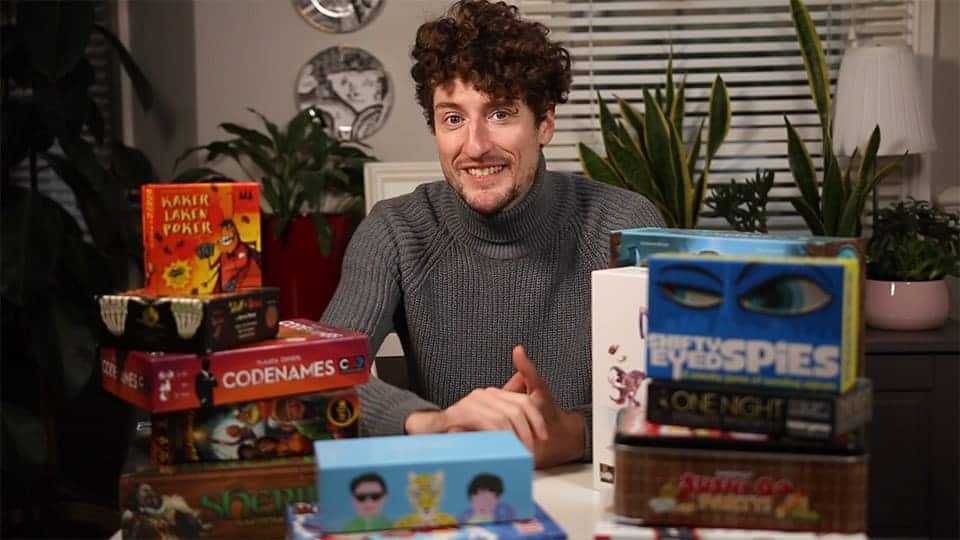In the photograph, a man with curly, dark, slightly disheveled hair and patchy facial hair is sitting at a table, smiling broadly at the camera, showing all his teeth. He wears a greenish-gray turtleneck sweater and has his hands clasped together. Behind him, there are various potted plants on tables against gray walls adorned with decorative plates and a window with white blinds. There's also a white lamp visible on one of the tables.

The main focus of the image is the collection of over 12 brightly colored board games spread out on the table in front of him. Notable games among them include Codenames, Shifty-Eyed Spies, One Night, and a Shrek-themed game, with one game featuring a red laughing beetle character. The man's bright eyes and joyful expression, coupled with the vibrant assortment of board games, create a lively and engaging scene.